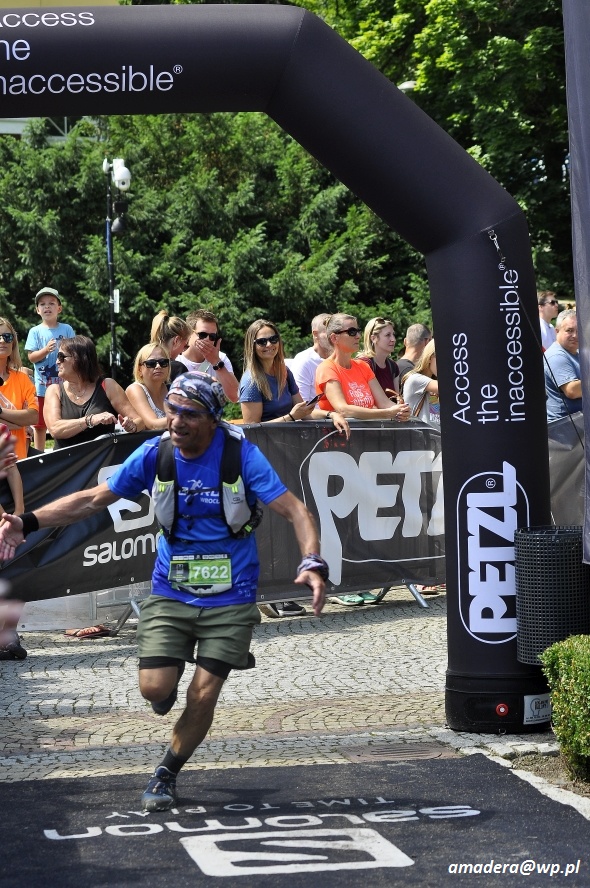In this detailed outdoor image, taken during the middle of the day, a runner is prominently featured at the center, crossing under a black finish line archway that reads "Access the Inaccessible" and "Pencil." The runner, appearing fatigued, is outfitted in a blue shirt, green shorts, running shoes, sunglasses, and a head covering. He also has a water backpack or vest on. The path beneath him is a concrete runway, possibly a stone path with painted markings. Behind the runner, a large crowd of spectators stands, separated from the track by a wall and a fence covered with a banner that also says "Pencil." The diverse colors in the image include black, white, gray, brown, tan, orange, light blue, green, red, highlighting various elements in the scene such as clothing and the surrounding environment. This picture encapsulates the lively and competitive atmosphere at the finish line of the race, capturing the anticipation and support of the spectators awaiting their loved ones' arrival.